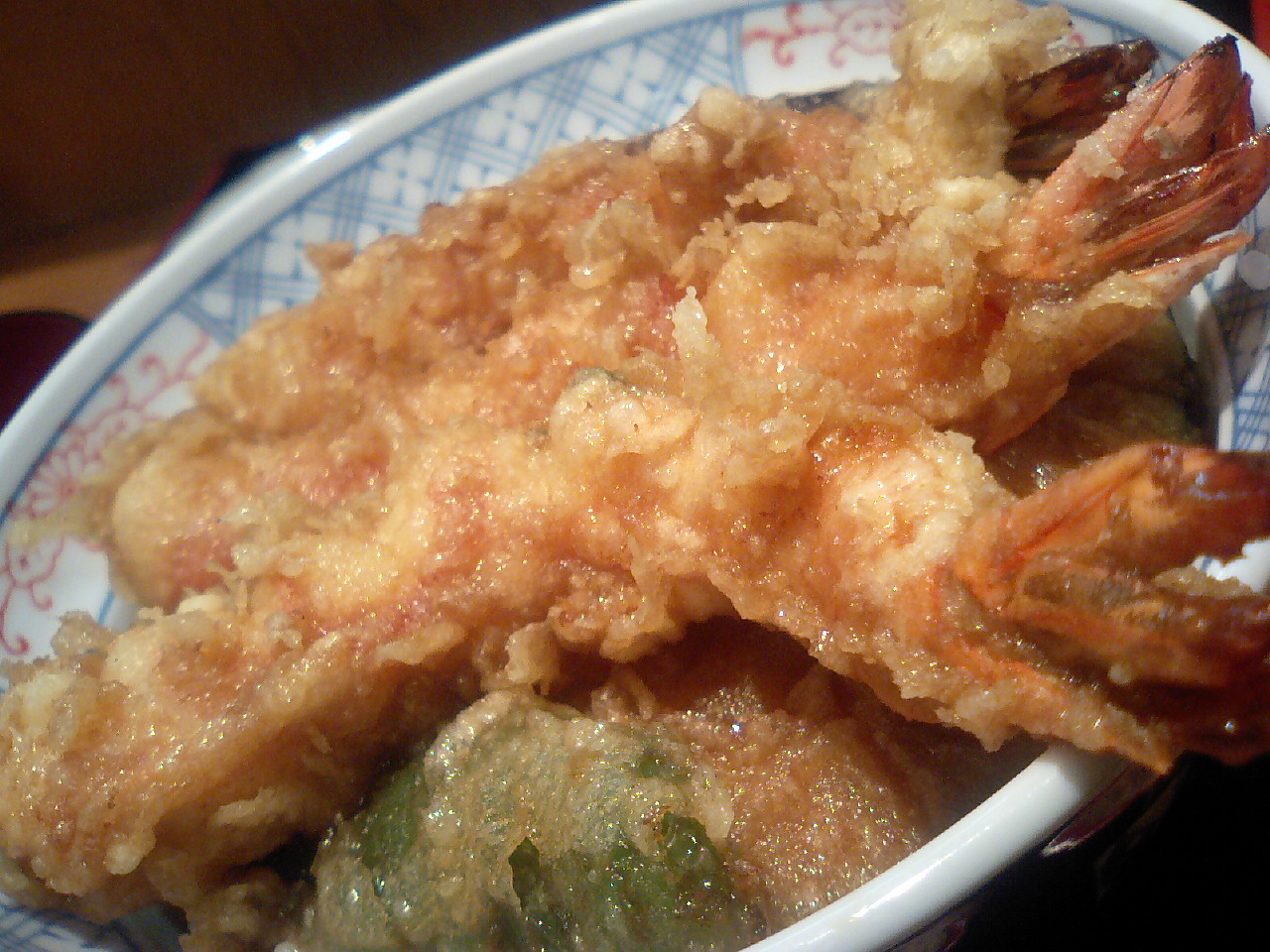The image showcases a close-up, landscape-oriented photograph of a dish featuring several large, breaded, and deep-fried shrimp, and some green, fried items possibly wrapped in wonton wrappers. The shrimp, appearing elongated with pink tails, are coated in a golden-brown breading that looks crispy and somewhat greasy. The food is arranged in an elegant shallow bowl adorned with blue checks, floral motifs, and red Asian symbols, hinting at a potential Asian cuisine influence. This detailed food presentation rests on what seems to be a restaurant table without any other dishes visible, enhancing the focus on the appetizing, glazed shrimp and their crispy green counterparts.